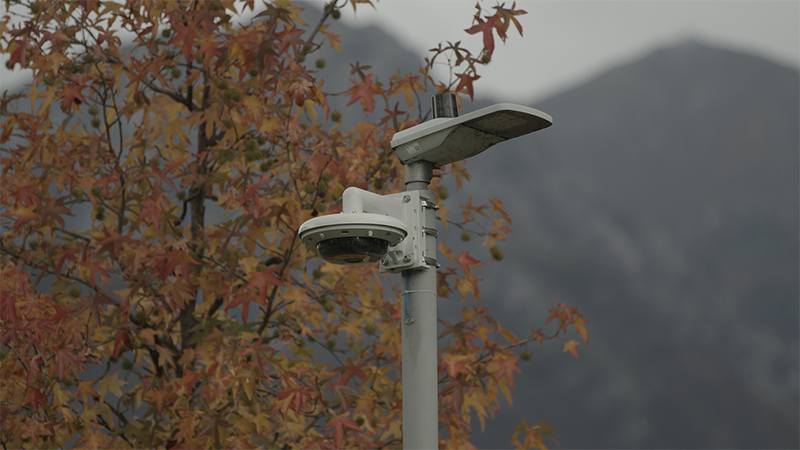The image captures a tall, slender light post with a gray metallic finish. Halfway up the pole, a horizontal white bar extends to the left, culminating in a downward-facing white circle, which appears to house a camera or sensor. Beneath this is a lighter gray circle, integrated into the pole, while at the top, a flat, black object projects to the right. Below this object is a barely visible light gray square that resembles a screen, with a silver pipe ascending from its upper right. To the left of the post stands a tree with a thin trunk and an array of leaves in hues of orange, light red, yellow, brown, and some green. In the background, a dark gray, blurry outline of a mountain is visible against a light gray sky, providing a serene yet somewhat obscured landscape.